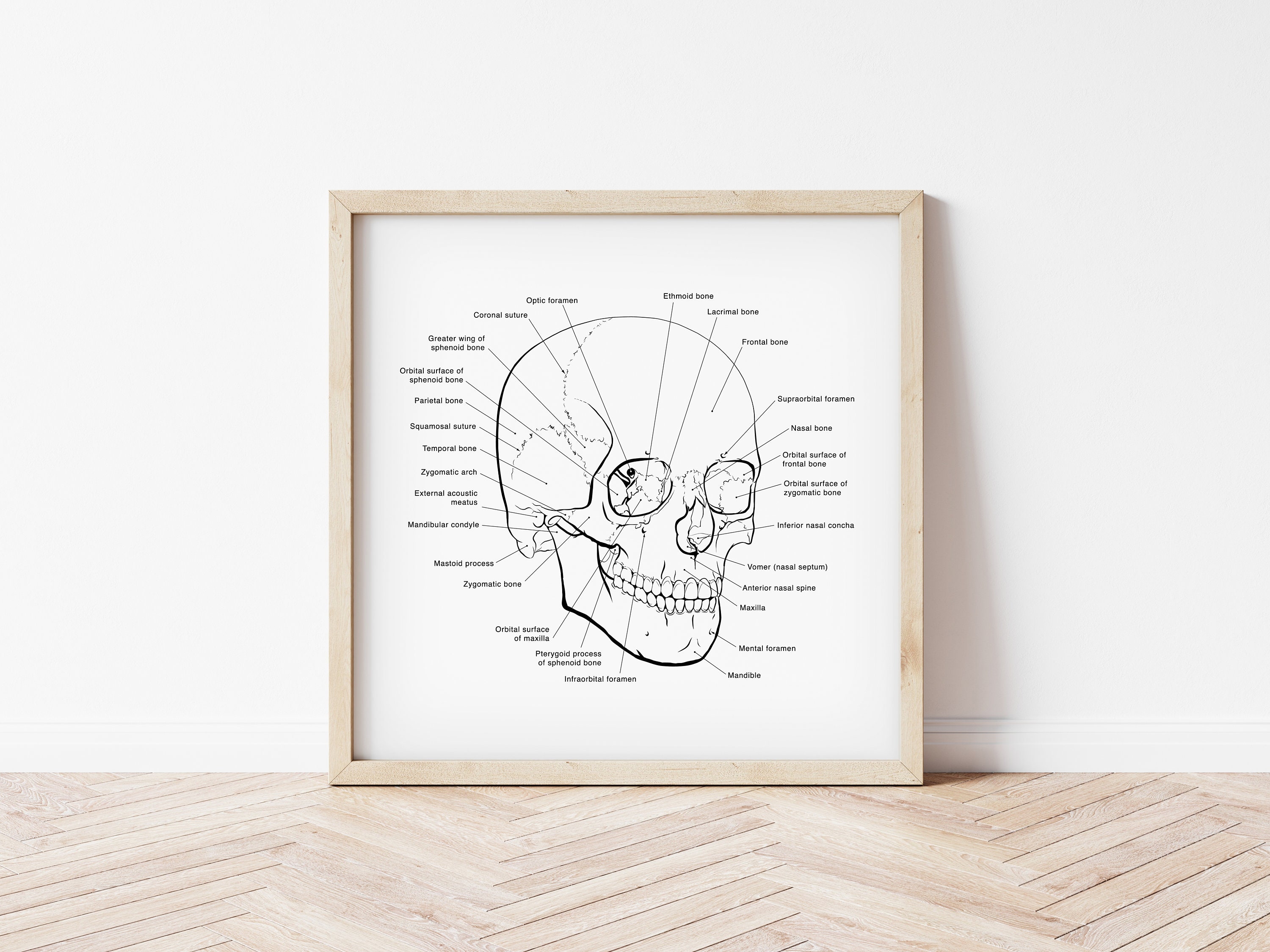This indoor color photograph captures a meticulously detailed anatomical illustration of a human skull. The illustration is rendered in black ink on white paper, depicting the skull in a three-quarter view with its jaw closed. The image is surrounded by numerous labels connected by lines, each pointing to various parts of the skull, providing a comprehensive guide to its anatomy—similar to what you would find in a medical textbook. This framed picture rests against an off-white wall, creating a stark background contrast that emphasizes the intricacy of the illustration. The frame itself is composed of light-colored wood, harmoniously matching the blonde parquet-style wooden floor beneath it, arranged in a houndstooth or V-pattern. The floor’s light wood and open-line grouts further accentuate the minimalist yet sophisticated setting of this educational artwork. The left-hand side of the image is brightly lit, while the right side casts a subtle shadow, adding depth to the overall presentation.